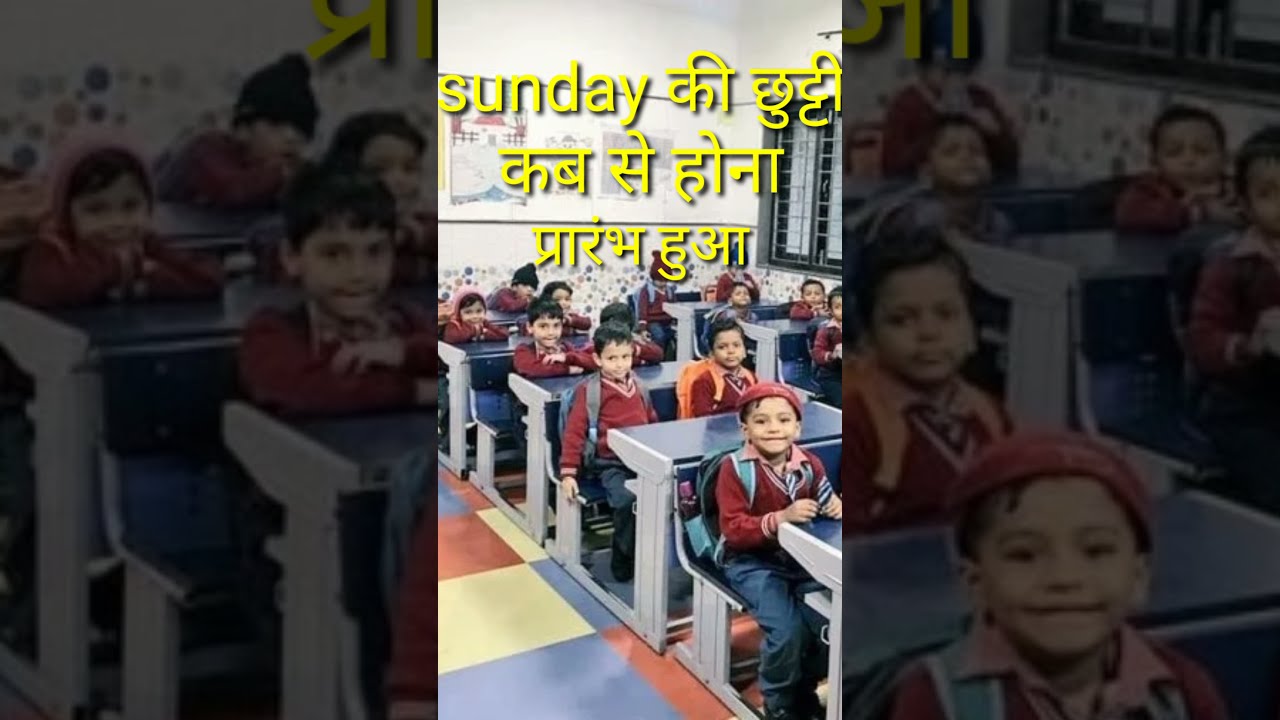This vertically-oriented cell phone photo shows a classroom likely in India or Pakistan, filled with young children approximately six or seven years old. The main image is centered with blurred and darkened edges expanded to fill the rectangular frame. There are 13 children, all boys, neatly seated in pairs at blue desks with gray sides that resemble booths. Each desk accommodates two students, creating an organized layout. The children are dressed in red maroon sweaters, blue pants, and some wear backpacks, suggesting they might be ready to leave or have just arrived. A prominent yellow caption at the top of the image reads "Sunday" followed by words in Sanskrit. The classroom floor features a vibrant pattern of red, blue, and yellow tiles, adding to the lively atmosphere. Many of the children are smiling directly at the camera, which is angled from the front of the room, capturing a cheerful and organized educational setting.